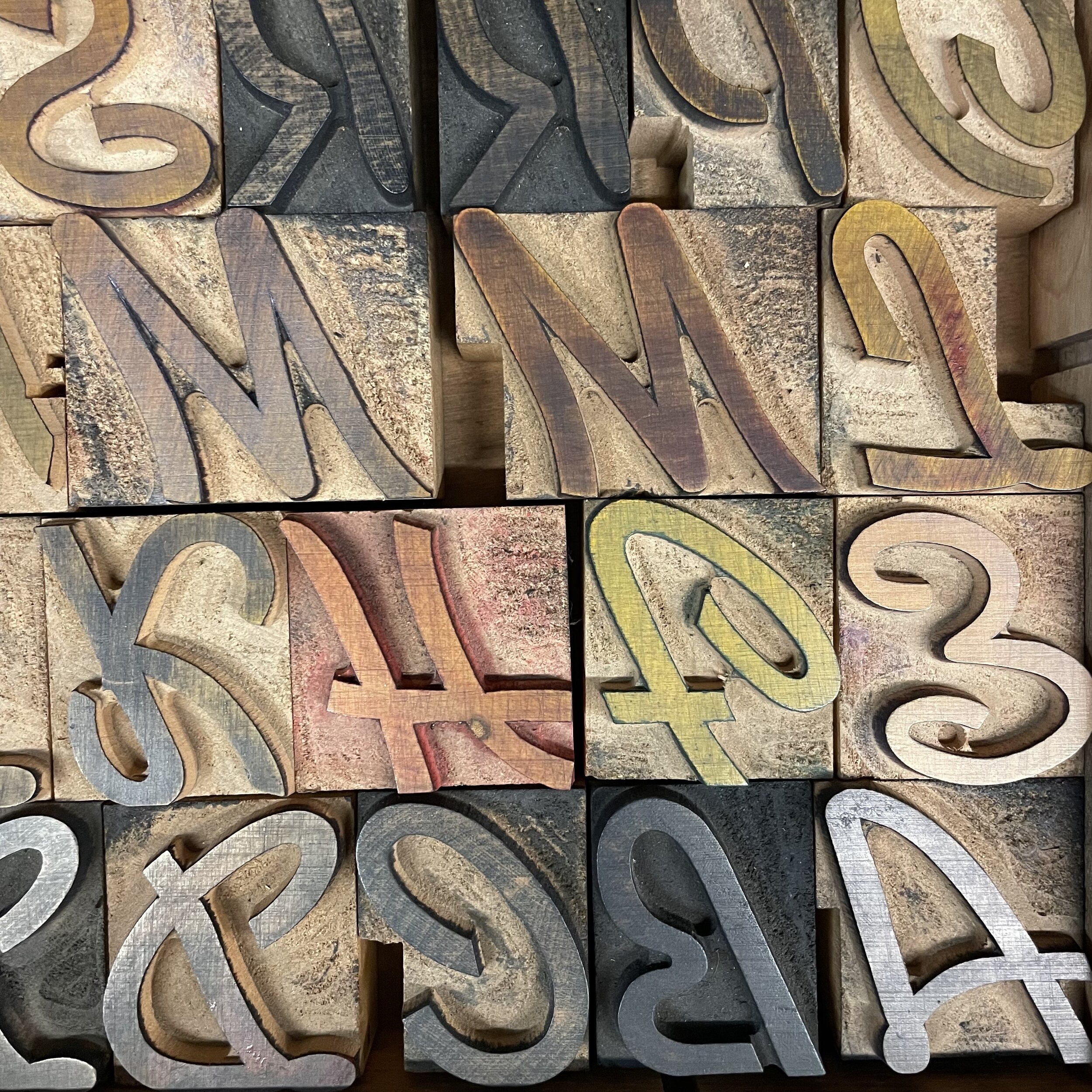The image showcases an array of wooden letter and number stamps, arranged in a tight, collage-like formation without any visible border, against a white background. The stamps are positioned face-down, allowing us to see a mirrored version of their engravings, which include a mix of letters such as A, B, C, D, F, H, K, L, M, P, R, S, W, and numbers like 3. Many of the stamps feature elegant, swirly script, suggesting they are part of a cohesive set. The stamps vary in color, exhibiting hues of natural wood, black, silver, yellow, brown, gray, and orange, with some showing signs of frequent use and darker ink residue, while others remain fresh and new-looking. There are four discernible rows: the top row, partially cut off; the second row showcasing M, M, L; the third row including K, H, F, 3; and the bottom row presenting D, C, B, A. The overall arrangement hints at the alphabet running in reverse order from bottom to top.